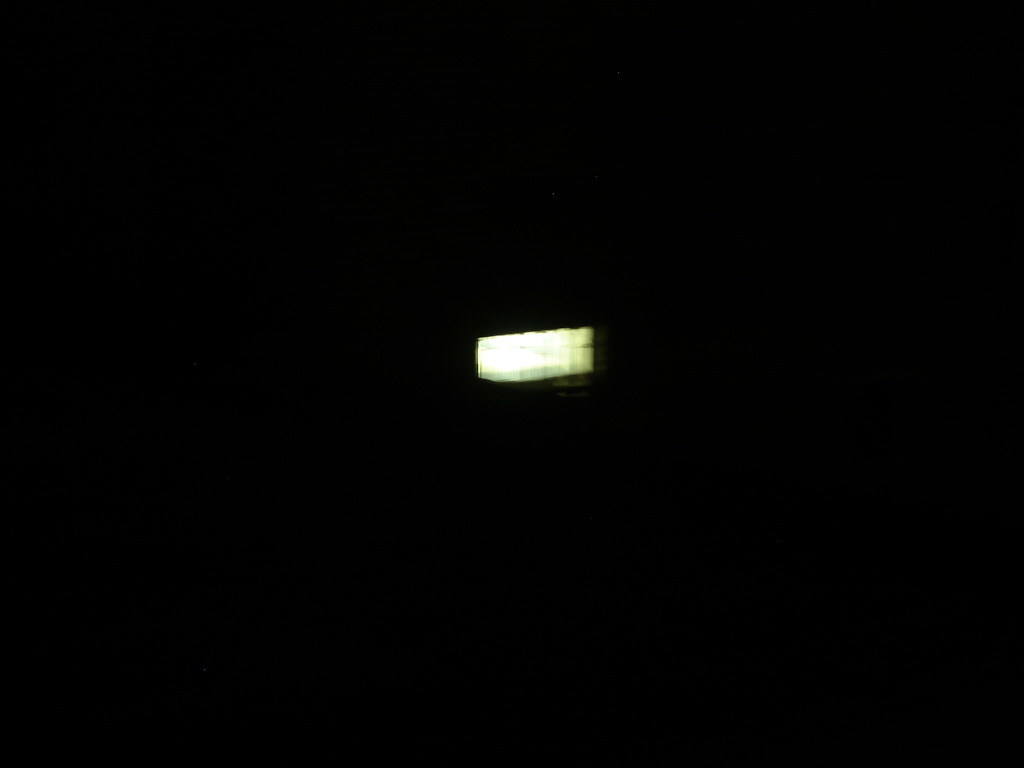In this nighttime photograph, an out-of-focus green LCD clock face dominates the center, occupying about a tenth of the image. The clock, a bright green blur, emits a soft glow against the otherwise impenetrable black background. Completely obscured by the blur, no numbers or text on the clock are discernible, resulting in a striking contrast between the vivid green light and the enveloping darkness. The overall effect is an abstract, almost ethereal impression of a clock, highlighted by the subtle, diffused green hue in the center of the frame.